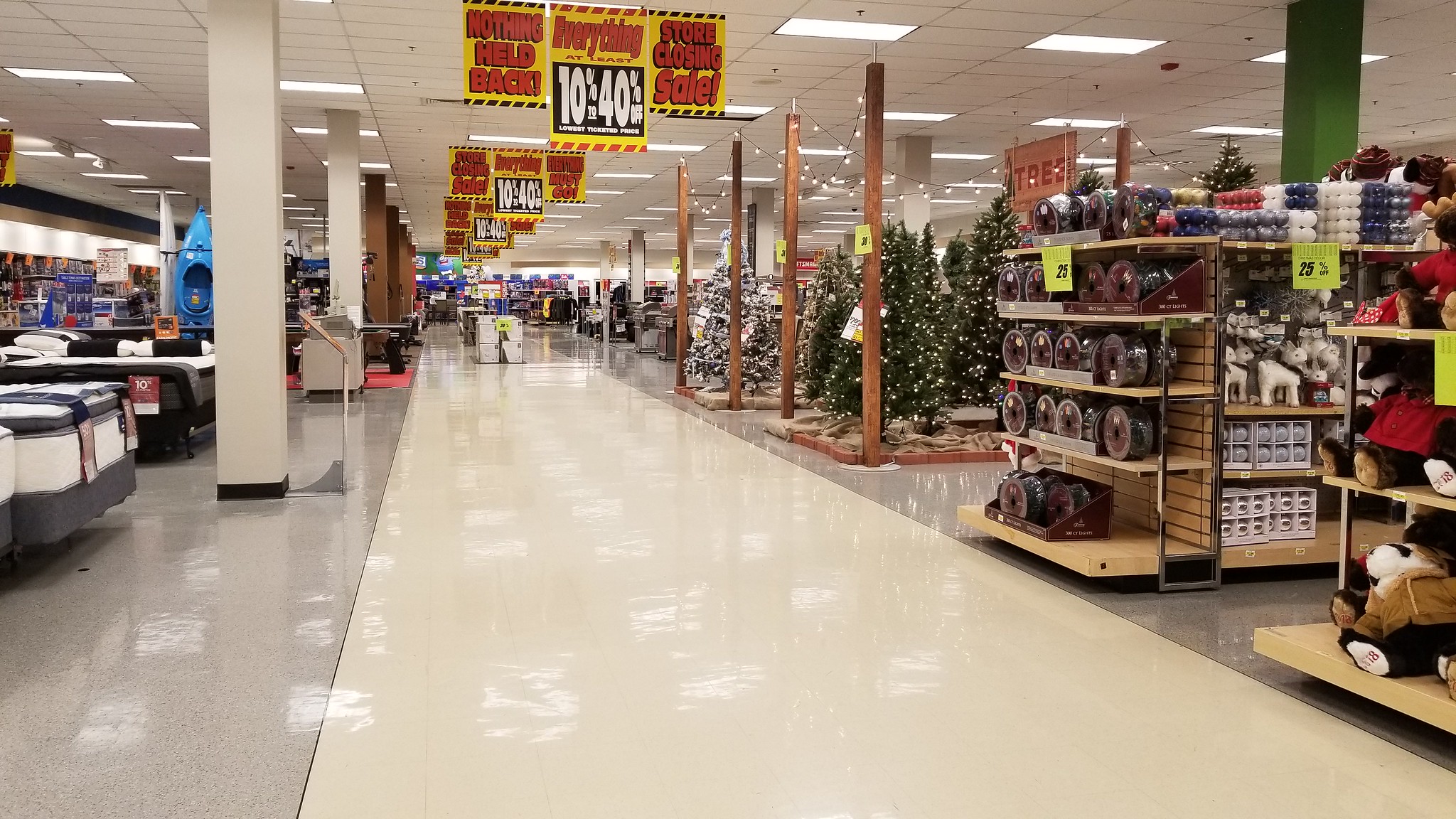The image depicts the inside of a large department store captured in a color photograph, vibrantly showcasing a festive and bustling retail space during the holiday season. The focal point of the image is a spacious aisle with a shiny linoleum floor, transitioning from white in the center to gray along the retail sections. Overhead, a white ceiling dotted with fluorescent rectangular lights illuminates the scene, casting reflections on the polished floor below.

Hanging from the ceiling, an array of bold yellow signs with red and white writing announce enticing sales and promotions, such as "10 to 40% off," "Nothing Held Back," and "Store Closing Sale." These signs extend down the aisle, drawing customers further into the shopping area. 

To the right of the aisle, festive Christmas decorations are prominently displayed, including tall, lit Christmas trees in black, white, and green, set upon brown stands and accompanied by wooden pillars. The shelves brim with seasonal items, perhaps small decorations and white reindeer figures, contributing to the holiday ambiance.

On the left, the edge of the image reveals white posts and what appears to be mattress sets, indicating varied product offerings that contrast with the festive décor on the opposite side. The wide assortment of goods and the bustling, decorated environment evoke a sense of holiday urgency, likely emphasizing a significant sale or clearance event in the store.